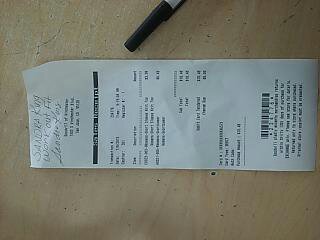The photograph depicts a receipt printed on traditional white paper with black ink, positioned sideways on a light, almost blonde-colored wooden tabletop. The tabletop itself shows signs of use, with visible scratch marks and darker black-colored holes. The text on the receipt is largely illegible due to its small size and the image clarity; however, at the top, it clearly reads "Sandra King Workout Fit" followed by "Sandra King." Above the receipt on the left side of the image, slightly off-frame, the black cap of an ink pen is visible. The receipt, indicative of a store register printout, includes a barcode at the bottom and various figures, though their specific details are unreadable.